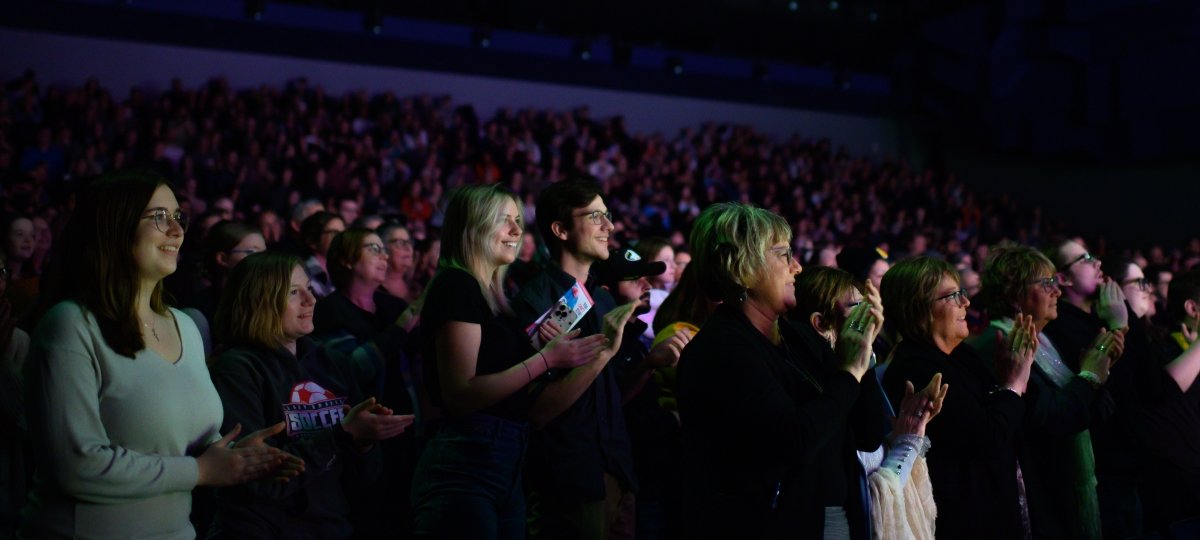The image captures a meticulously ordered audience attending a show or concert. The attendees are neatly arranged in rows and aisles, all uniformly facing towards the stage, which is the sole light source in the scene. This illumination highlights their faces and the front of their bodies, casting the rest into shadow. The crowd predominantly consists of older white women, suggesting that the performer or event is one that resonates particularly with this demographic. The overall atmosphere is one of focused anticipation as the audience is enveloped in the soft glow from the stage.